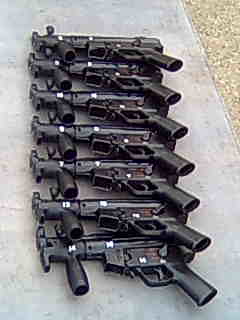In the photograph, there's an arrangement of seven black submachine guns, identified as MP5s, neatly stacked on top of each other. These guns, each equipped with a front handgrip and an ammunition clip positioned in front of the trigger, are laid out in a vertical line formation. The photograph appears to be taken outdoors on a light-colored, white pavement or cement flooring, with a small patch of yellow gravel visible to the side. The scene is illuminated by natural, albeit overcast light, indicating a cloudy day. There are no people or additional objects in the image, just the neatly arranged firearms on what seems to be a rough aggregate floor.